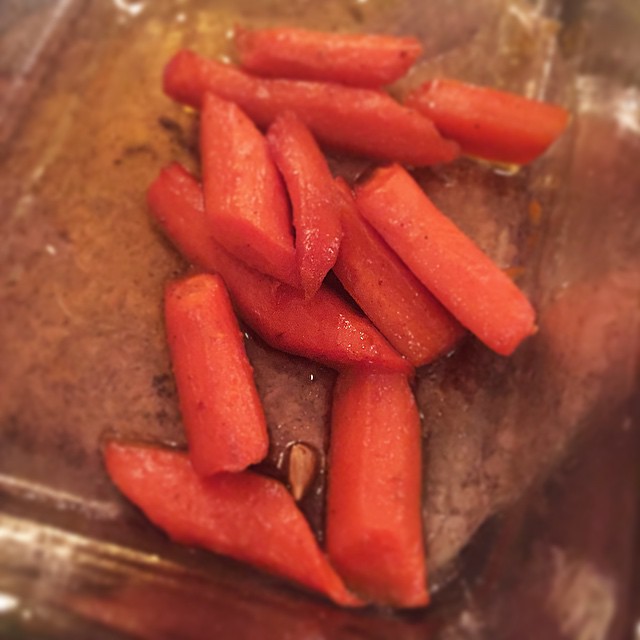This image shows a blurry, close-up photograph of what appears to be cooked baby carrots or possibly thin-sliced red peppers, all cut into elongated, cylindrical pieces about an inch long. The food, deep reddish-orange in color, glistens with a coating of oil or butter, suggesting it could be either roasted, sautéed, or steamed. The items are irregularly chopped with the ends cut diagonally, resting in what seems to be a glass or metallic dish, as indicated by the light reflections on its sides. Amidst the juicy-looking slices, a visible lemon seed can be seen in the bottom center. The photograph is dark and of poor quality, with no text or date stamps, offering a down-angled view, capturing less than half of the dish.